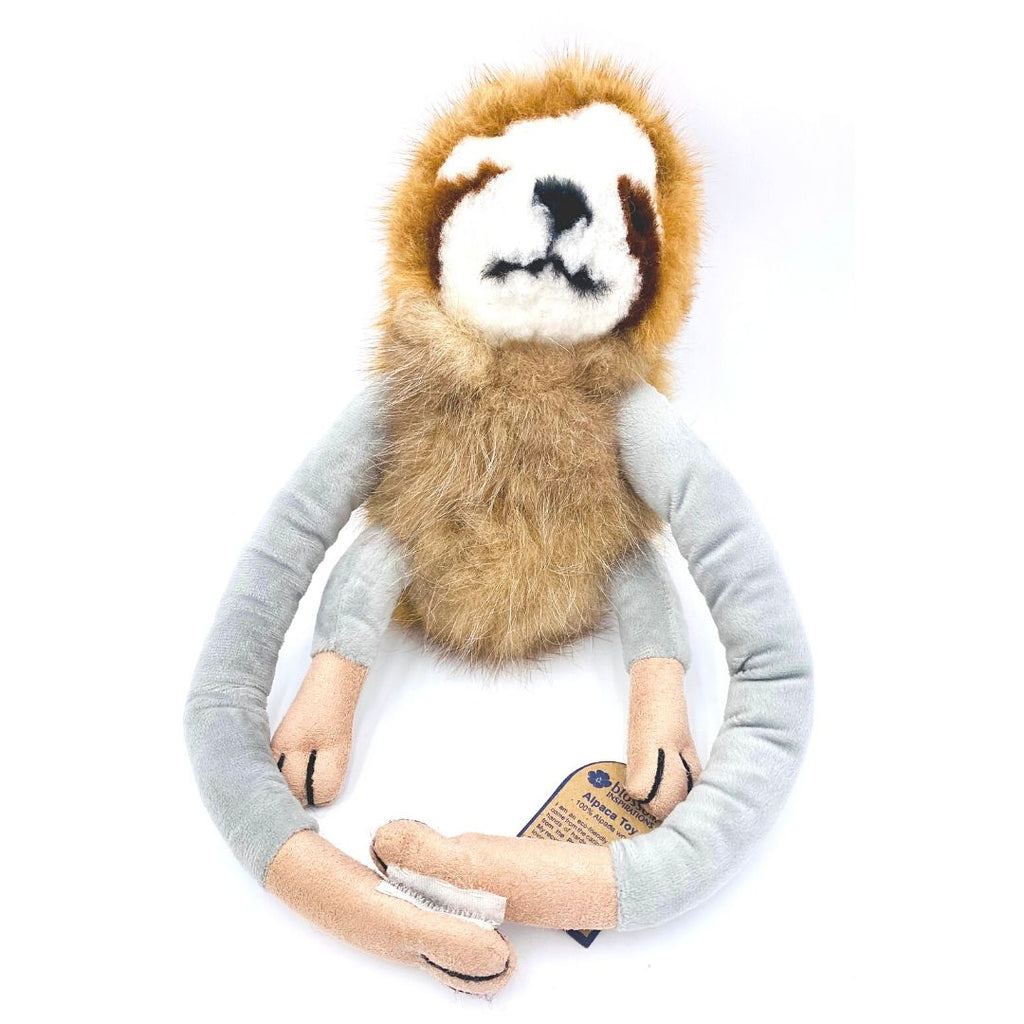This image features a stuffed animal with a light brown, fuzzy body and a white face adorned with brown patches around its eyes. The nose and mouth are black and form a single piece. The face is bordered by a halo of slightly darker brown fur. It convincingly resembles a sloth, complete with two very long, gray arms that extend in front of it, ending in peach-colored hands that have Velcro, allowing the arms to wrap around objects or oneself. The stuffed animal also has two much shorter gray legs, ending in peach-colored feet. There is a small label attached to one of its feet, which reads "100% alpaca toy," adding a peculiar detail, as the toy itself clearly mimics a sloth. The background of the image is white, drawing attention to the unique and charming details of the toy.